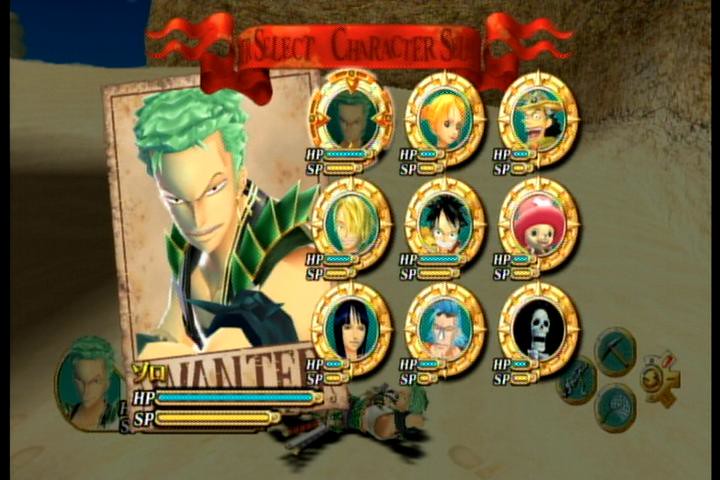This is a detailed caption formulated for the described image:

---
A screenshot from a video game adaptation of the "One Piece" anime and manga series, featuring a character selection screen. The interface has a brown background with a prominent red banner at the top that reads "Select Character." The focal point of the screen is a highlighted character whose portrait is displayed on a "Wanted" poster to the left. This character, drawn in the distinctive anime style, has green hair and his name written in Japanese. Below the portrait, the poster is emblazoned with the word "Wanted." Additionally, the screen shows the character's hit points bar and special powers bar. Other selectable characters are also visible, including the protagonist Monkey D. Luffy, the adorable Tony Tony Chopper, and a skeleton-like character likely to be Brook.